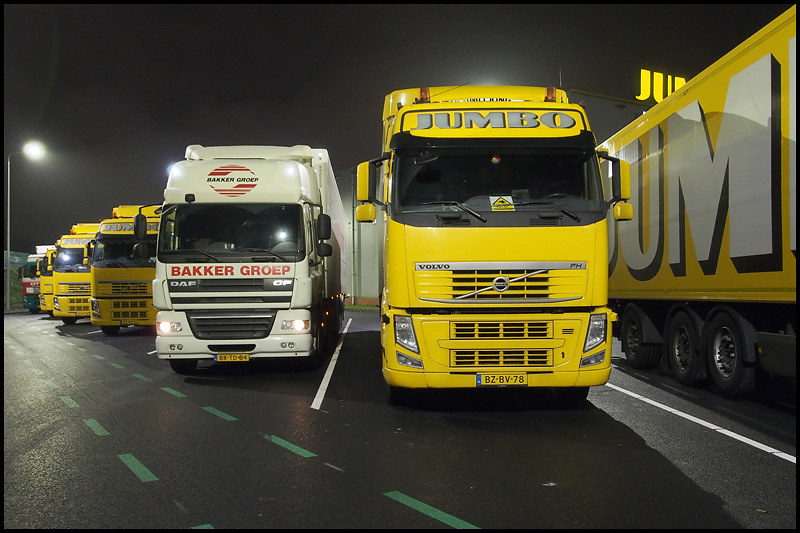The image depicts a nighttime scene in a European parking lot filled with several large tractor-trailer trucks. Prominently featured are six trucks lined up in a row on black asphalt, each parked within marked lines, with green and white dashed lines on the pavement indicating parking alignment. The yellow trucks, all sporting the word "Jumbo" in silver writing and bearing European license plates, are identified as Volvo trucks. In contrast, there is a white truck, distinguished by red writing that says "Bachergruppe" (or "BAKKER GROEP" as noted in one caption). The trailers of these trucks are visible, with one yellow trailer displaying the letters "UM" boldly. Despite slight variations in truck colors, the consistent presence of the "Jumbo" branding and the organized arrangement under faint artificial lighting highlight a sense of orderly commerce in this darkened parking lot.